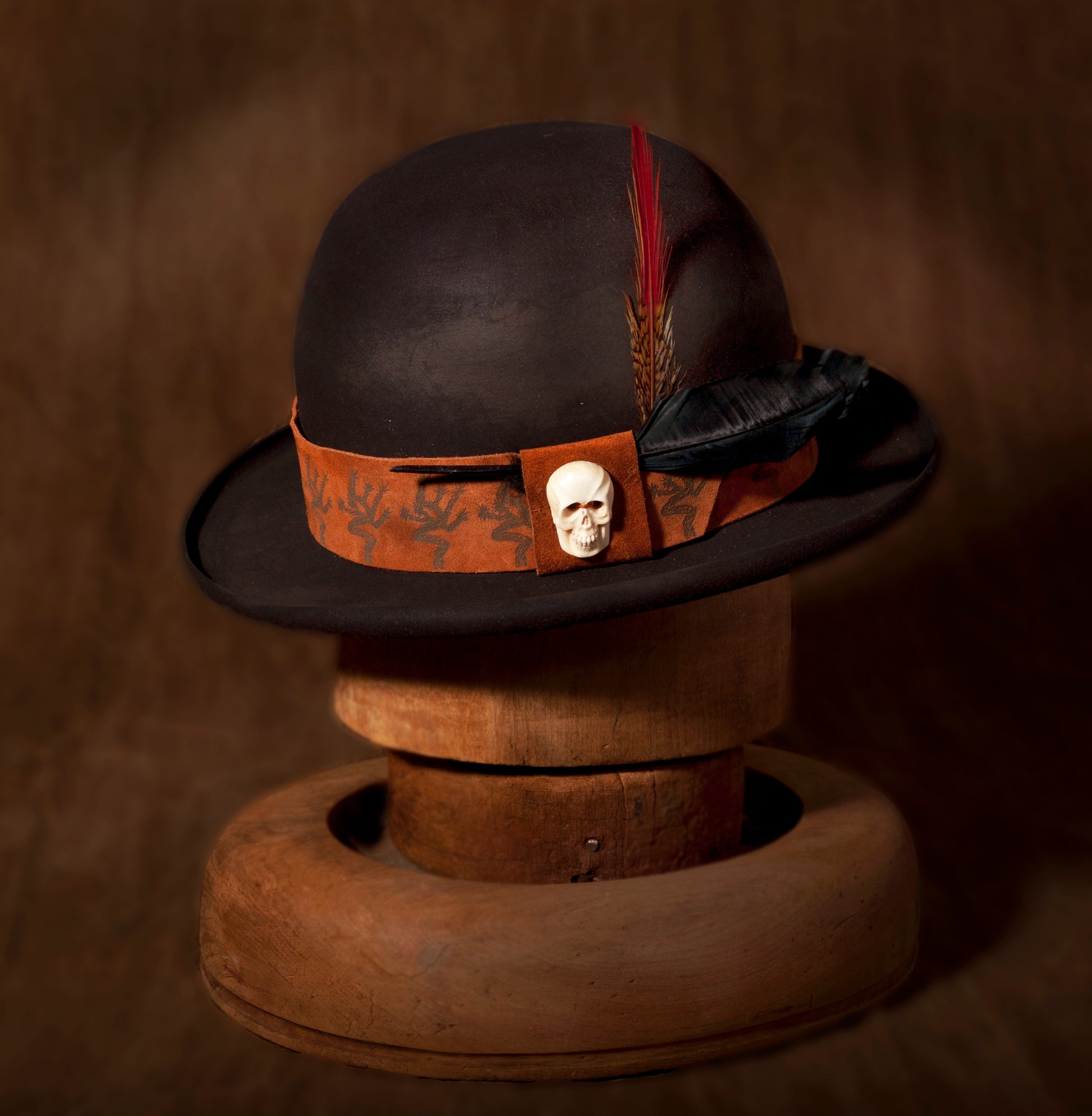The image depicts a dark brown, brimmed hat, reminiscent of a bowler or derby style, placed on a wooden hat stand. The stand features a circular base with a cylindrical extension in the center to support the hat. This stand, crafted from wood, has a rustic appearance. The hat itself is adorned with an orange ribbon encircling the brim. Prominently placed on the ribbon is a white, plastic skull. Extending from the ribbon are two feathers: a red feather with a brown base situated vertically, and a black feather positioned horizontally. The background of the image appears dark brown and shadowy, suggesting the hat and stand are placed on a table. Notable shadows accentuate the upper right, upper left, and particularly the bottom right middle sections of the image, adding depth and contrast to the scene.